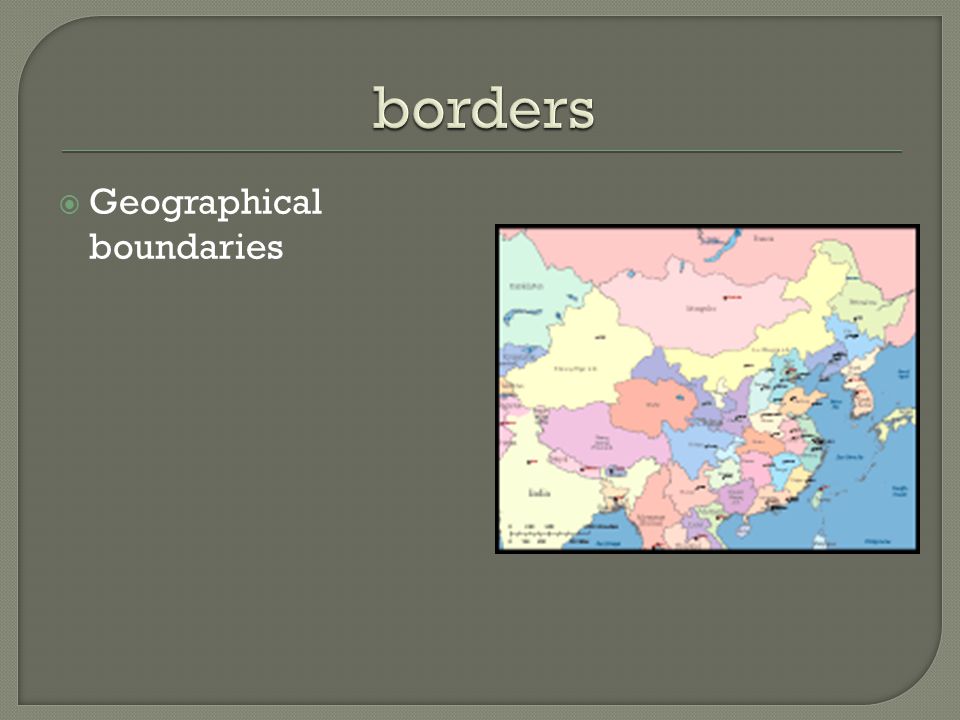The image is a PowerPoint slide predominantly featuring a map of a specific region of the world. The slide has a structured layout with a lighter gray border and a darker gray center, creating a sharp-angled look on the lower left and upper right sides, with a curved design on the upper left and lower right corners. At the top, “Borders” is written in white letters, with a teal underline beneath it. Directly below, on the left side, there is a green bullet point followed by the text "Geographical Boundaries" in white. 

The map, which occupies the right side of the slide and is slightly off-center, is colorful and detailed. Although the names of the countries are too small to read, the map includes various shades of gray, pink, lighter pink, pastel green, pastel blue, dark blue, yellow, purple, and orange. The ocean is depicted in blue and is positioned on the right side of the map. The background of the slide is notably sparse, implying an educational setting designed to teach about geographical regions and boundaries.

The overall slide design emphasizes a clean, educational aesthetic, with clearly marked sections and vibrant colors to differentiate between geographic and political features.